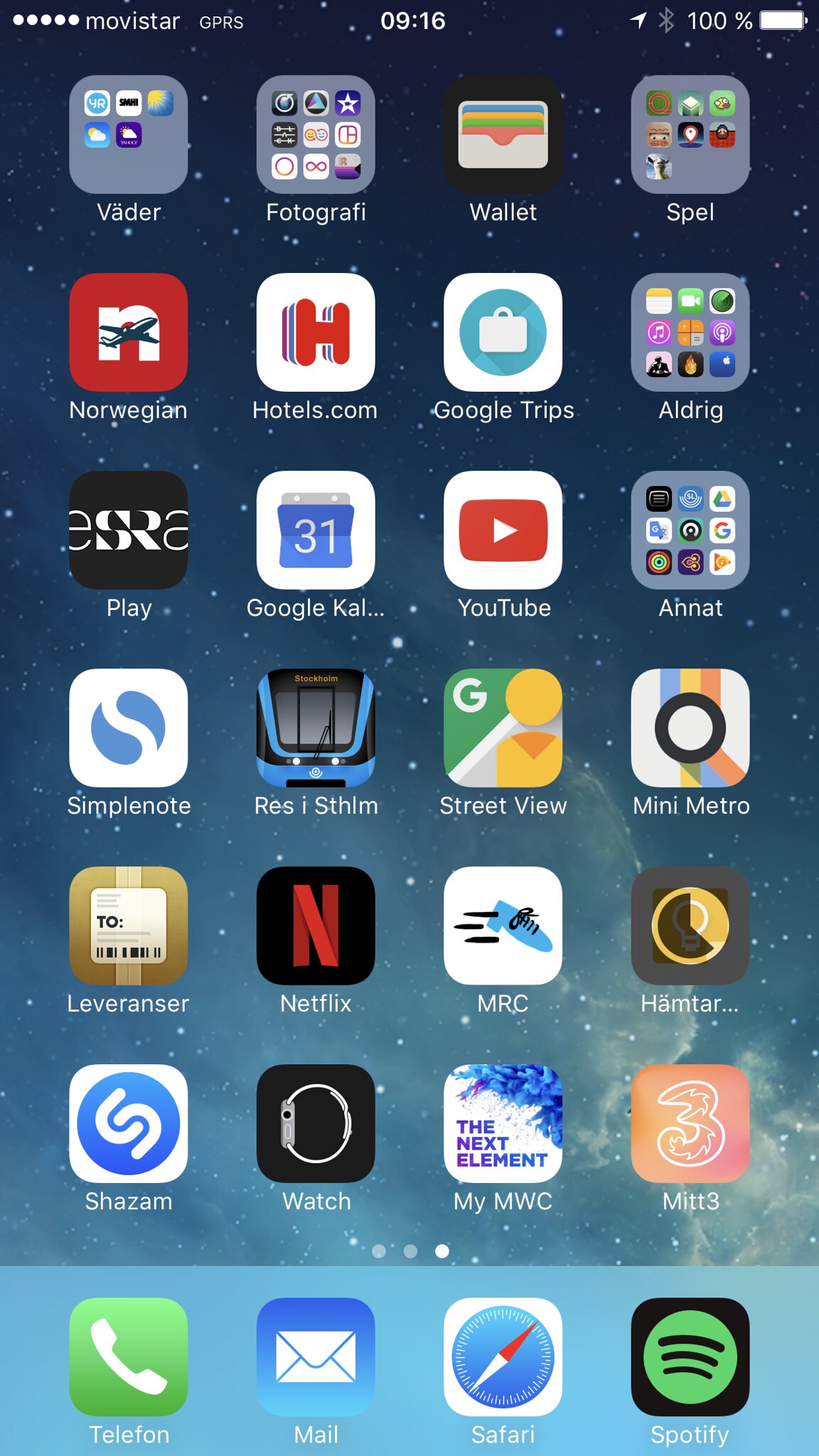This image captures a detailed screenshot of a smartphone home screen featuring a variety of app icons arranged in a grid on a night sky-themed background. At the top of the screen, the status bar reads "MovieStar GPRS" and shows the time as 9:16 with a battery life at 100%.

The apps are organized in a 4x6 grid, spanning six rows. In the first row from left to right, the apps displayed are Vader, Photography, Wallet, and Spell. The second row features Norwegian, Hotels.com, Google Trips, and Aldridge. The third row shows Play, Google Calendar (Google Cal), YouTube, and Anat. The fourth row contains Simple Note, Resi, Sysilm, Street View, and Mini Metro. In the fifth row, apps include Lever Answer, Netflix, MC, MRC, and Hamatar. The sixth row lists Shazam, Watch, MyMWC, and MIT3.

Beneath this grid, a lighter blue section holds four essential apps: Telephone, Mail, Safari, and Spotify. The entire home screen sits against a dark blue, star-studded night sky, transitioning to a lighter blue at the very bottom.